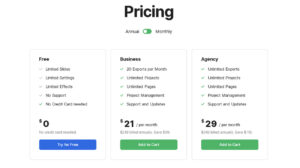Here is a cleaned-up and detailed caption for the image based on the provided voice description:

---

The image features a pricing table set against a white background. At the top and center of the image, the word "Pricing" is prominently displayed in bold, large black font. Directly underneath this title, the content is blurry and unreadable. On the left side of the image is a black-colored word, possibly indicating a plan type, illustrated next to an oval shape. The oval shape resembles a battery icon, which is white on the left side and green on the right side.

The image appears to present three distinct pricing packages. The first package features the word "Free" at the top in bold. Below this, a list of five features or attributes is noted in black font, though the specific items are not legible. At the bottom of this section, it states "zero dollars" in black, followed by a blue rectangular button with the words "Try for Free" in white font.

The second package has a bold word at the top, which is not recognizable. However, it includes the price "$20 per month" clearly displayed. There is also a green rectangular button beneath the price, with the white font being unreadable.

The third and final package appears to be labeled "Agency." Although the rest of the content in this section is blurry and unreadable, the price listed is "$29."

---